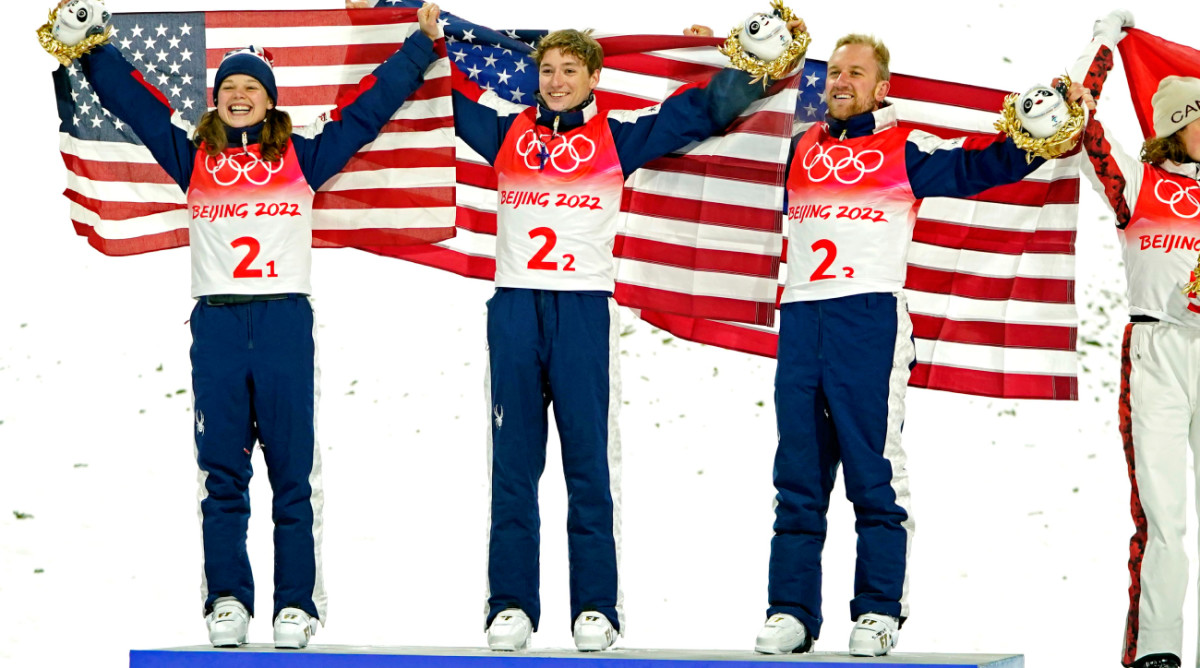This is a photo from the Beijing 2022 Olympics featuring four members of Team USA. Each athlete is proudly holding an American flag behind them and wearing a red and white vest over blue pants and jackets. The vests display "Beijing 2022" in red letters, Olympic rings, and numbers ranging from "21" to "24". The two women flanking the group—a woman on the left in a blue beanie and another in a white sweatsuit—and the two men in the middle, are all holding gold wreaths containing a panda stuffed animal. The athletes' triumphant expressions and the shared elements of their uniforms and flags highlight their unity and victory.